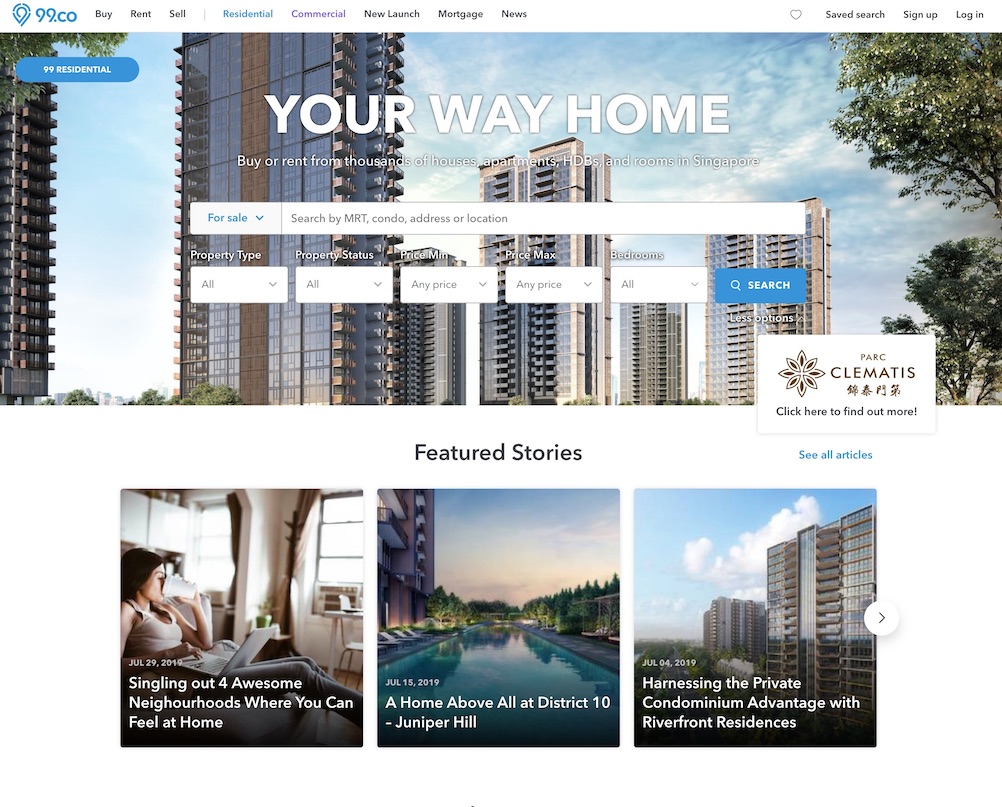The top of the page features a colorful banner showcasing a skyline filled with numerous corporate buildings in the city. Centered prominently within the banner, bold white text with a thin black border reads "Your Way Home." Below this, a subtitle in clean, legible font advertises, "Buy or Rent Thousands of Houses, Apartments, HDBs, and Rooms in Singapore."

Beneath the text, an interactive search field invites users to "Search by MRT, condo, address, or location," displayed in subtle gray text within the editable field. 

To the left of the search bar, a small bold blue font labeled "For Sale" accompanied by a downward arrowhead indicates a drop-down menu. Adjacent to this, a label reads "Property Type" with a drop-down menu set to "All." Following this, another field labeled "Property Status" also equipped with a drop-down menu set to "All." 

Continuing the sequence, fields for "Price Min" and "Price Max" both offer drop-down menus set to "Any Price." Lastly, a "Bedrooms" drop-down menu displays "All."

To the immediate right of these search filters, a medium blue background icon features the word "SEARCH" in bold, white capitalized text, accompanied by a small magnifying glass icon.

In the right corner of the banner, a distinguished logo resembling a lotus flower in brown color can be seen. Next to it, the text "PARC" is displayed in brown capital letters, followed by the larger text "CLEMATIS" in the same font. Below the logo, there are some characters in Chinese or Japanese, and a call-to-action message reads, "Click here to find out more."